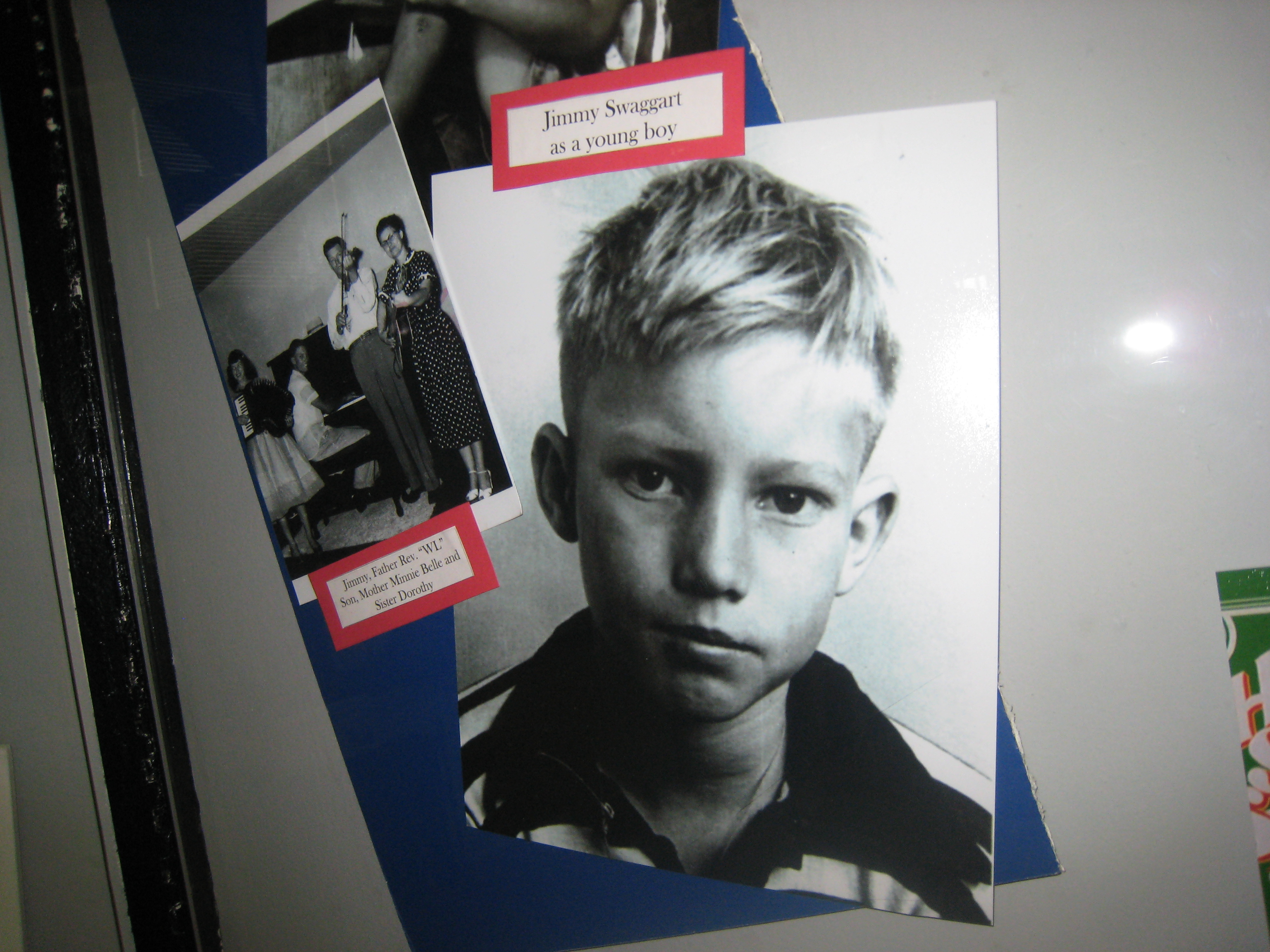The image is a detailed photograph of a photo montage posted on a white reflective dry erase board. The edges of the board, black and prominent, frame the scene. At the center of the montage, the largest and most striking image is a black-and-white portrait of a young Caucasian boy, likely around 6 to 8 years old, with short blonde hair and a polo shirt. Above this image, a typewritten caption on white paper with a red border reads, "Jimmy Swaggart as a young boy." 

To the left of this central photograph, there's another black-and-white image of four people engaged in a vibrant musical performance. This smaller picture shows a woman with a guitar, a man with a violin, a person with a piano, and another woman playing an accordion. Below this image, another red rectangular caption with white center reads, "Father Rev W.I. Sin Mother Minnie Bell and Sister Dorothy."

At the top of the board, a third black-and-white photograph is nearly cropped out, showing just a set of legs. Additionally, at the bottom right of the montage, partially obscured by the central image, is a green piece of paper with white lettering. The entire composition captures a nostalgic and intimate glimpse into the past, emphasized by the reflective qualities of the dry erase board and the subtle flash glare from the camera.